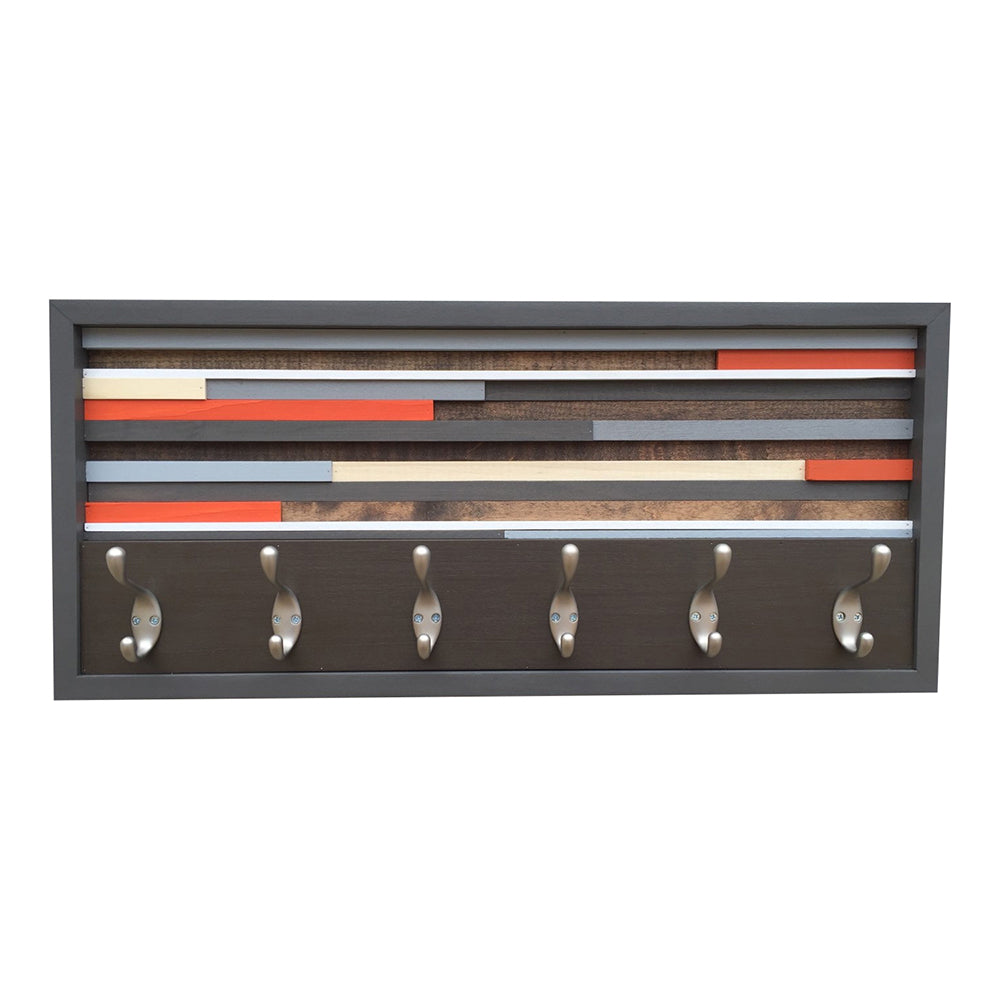The image depicts a horizontal, rectangular coat rack featuring six silver hooks attached to a dark brown wooden panel. Set against an edited-out white background, this product photograph creates the illusion of the coat rack floating in an empty void, drawing full attention to the item itself. A dark frame surrounds the entire piece, enhancing its prominence.

In the lower section, six hooks are arrayed along the bottom, each hook secured by two screws into the wooden panel. Above the hooks, the top half of the coat rack showcases a decorative inlay of various horizontal stripes in an artistic, seemingly random pattern. These horizontal lines include an incomplete red stripe at the top, followed by a solid white stripe. Below these are gray and additional red stripes, with another stripe featuring blue at one end, red at the other, and white in the middle. Additional horizontal lines in varied colors like light gray, dark gray, brown, orange, and black complete the intriguing design. The overall palette of the coat rack includes shades of gray, brown, white, blue, and red, contributing to its detailed and visually appealing aesthetic.